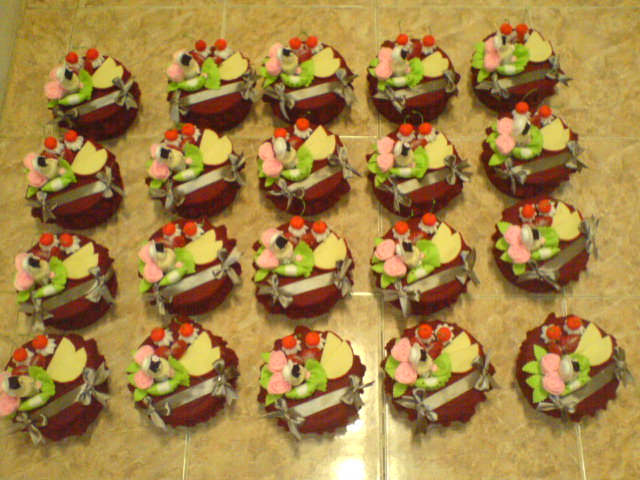In this blurry, color snapshot photograph, an arrangement of 20 intricately decorated pastries—possibly cupcakes or mini cakes—are laid out in four rows of five on a tan or reddish-tinted tiled surface. Each pastry features a scalloped edge with a dark chocolate base and is adorned with various decorative elements, including pink flowers, rose-like designs with leaves, cream-colored half-moon shapes, red dots, lemon or lime slices, strawberries, raspberries, and green garnishes. The overhead kitchen light casts a noticeable yellowish-orange hue particularly towards the lower part of the image, enhancing the vibrant decorations on the pastries. The arrangement is shot from an overhead perspective, emphasizing the neat rows and meticulous detailing on each treat.